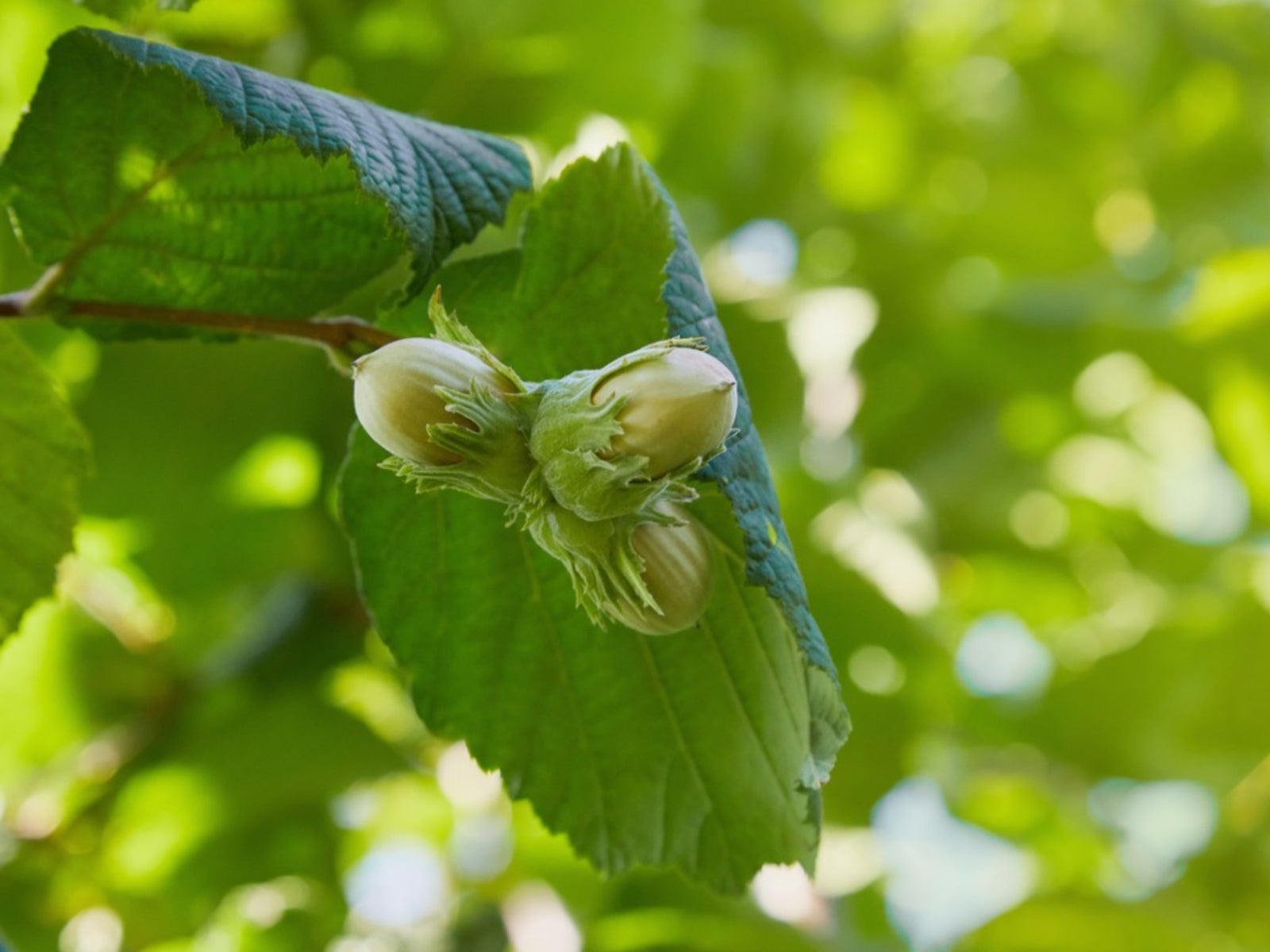This wide, outdoor photograph captures a close-up of the end of a tree branch, prominently featuring a cluster of developing seeds. Emerging from the left side of the image, the main branch supports three large green leaves, with the largest leaf positioned centrally within the frame. Just in front of this dominant leaf, three seed-like objects—pale yellowish to off-white in color and resembling acorns—are firmly attached. Small green vegetative parts encircle their tops. The seeds appear robust and not yet ready to fall. The background, bathed in daylight, displays out-of-focus tree leaves, enhancing the image's focus on the branch and its budding seeds. Sunlight softly reflects off the leaves, adding a gentle glow to the scene.